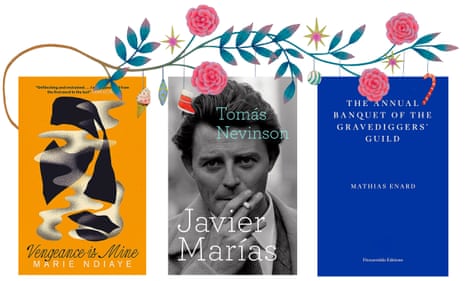The image displays three book covers against a white background. On the left is an orange book cover titled "Vengeance is Mine" by Marie NDiaye. This cover features intricate black and white squiggly designs that resemble abstract forms, possibly a fragmented image, with "Vengeance is Mine" in black text and the author's name in white text. In the center, there is a book titled "Tomas Nevinson" by Javier Marías, featuring a black and white photograph of a man with dark hair smoking a cigarette. On the right, the book titled "The Annual Banquet of the Grave Diggers Guild" by Matthias Enard is shown. This cover showcases a branch adorned with four pink roses, along with various whimsical items such as a candy cane, Christmas stockings, an ice cream cone, and a green and white striped Christmas ornament.